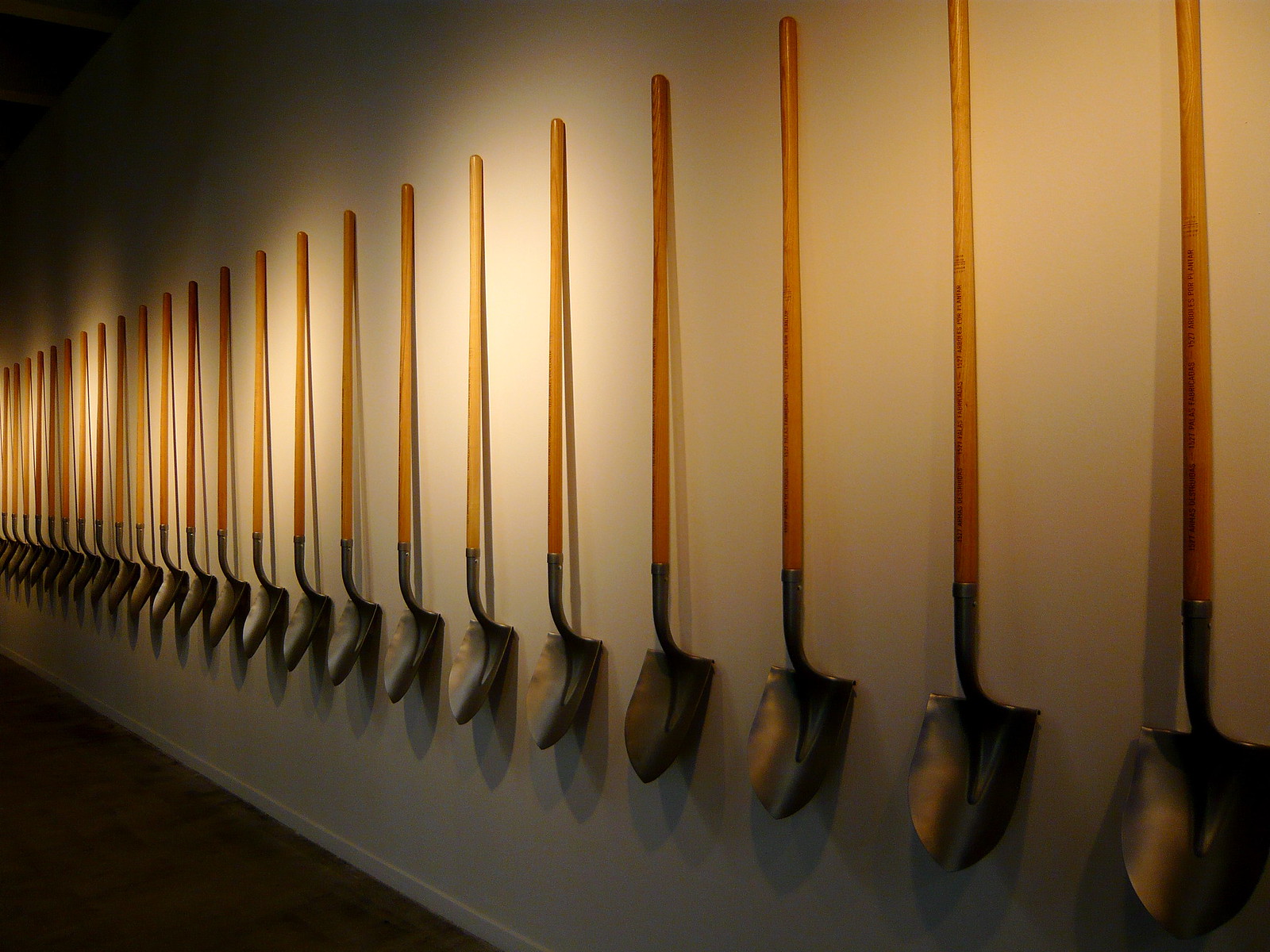The image showcases an art installation of brand-new shovels meticulously mounted on a white wall. Each shovel, with its light wooden handle and chromey-silvery blade, is evenly spaced both horizontally and from the floor, creating an orderly display that spans from one edge of the photograph to the other. The lighting, reminiscent of museum spotlights, casts multiple shadows of the shovels on the wall, adding a layered visual effect that makes the tools appear to multiply as they recede into the distance. The room itself is dimly lit, with the primary focus being the shovels, which seem to glow under the directed lighting. The setting suggests a museum or exhibit space, with the hardwood floor in the foreground and the neutral-toned wall enhancing the simple yet striking composition of the installation. There are at least 20 shovels visible, giving a sense of endless repetition as they appear to diminish in size down the wall due to the perspective.